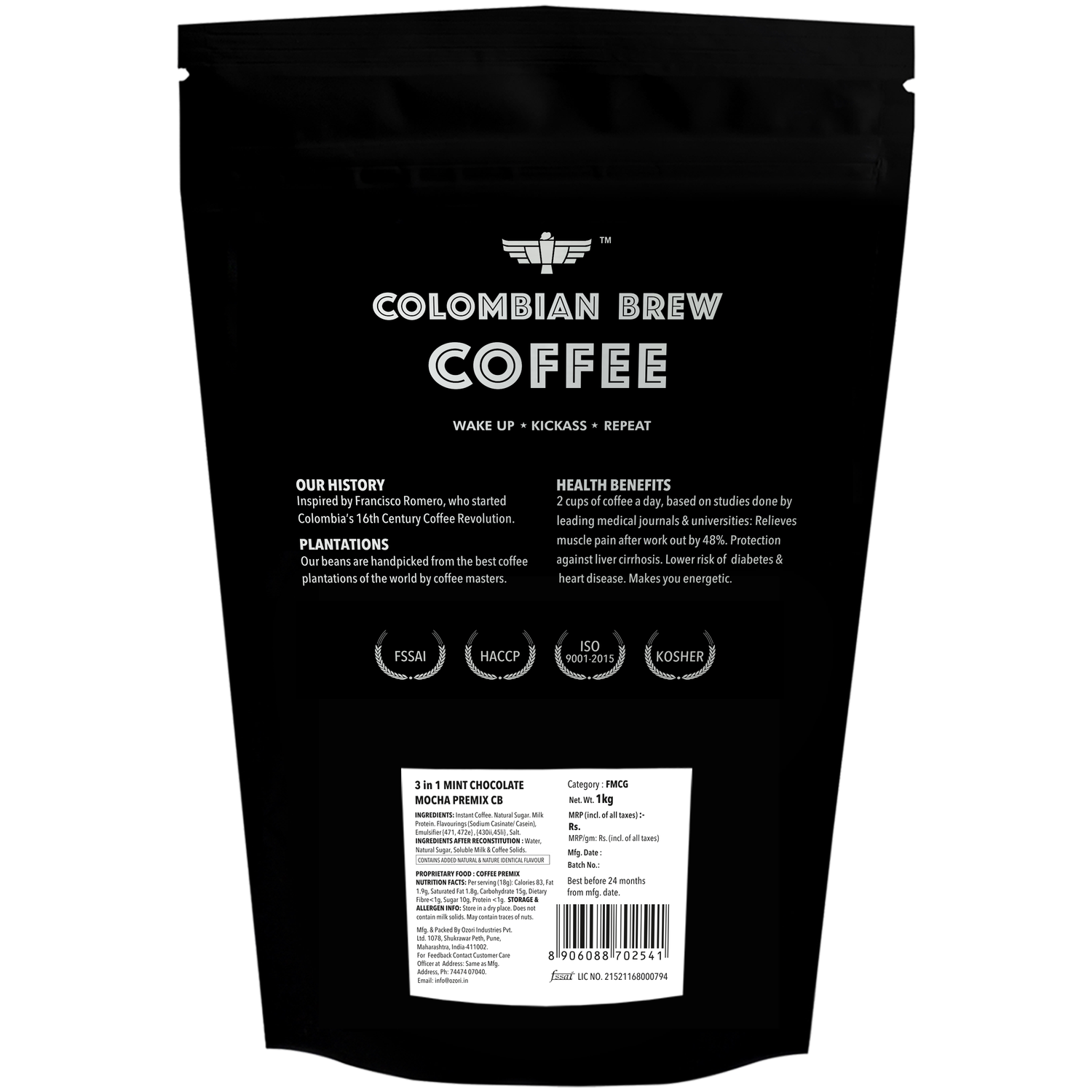The image presents a vertically oriented, rectangular black bag of coffee standing upright against a white background. Adorned with white font and images, the bag prominently features a Native American Thunderbird logo with a trademark symbol. Above, the text "Colombian Brew Coffee" is inscribed in white, followed by the bold slogan "Wake Up, Kick Ass, Repeat." Beneath these elements, multiple sections of small white text are visible, though difficult to read; they are labeled "Our History," and "Health Benefits," with mention of "Plantations." On the left side, there are several certification seals, including "Kosher," "HACCP," and "FSAI," all encircled in gray. At the bottom, a white nutritional label is visible, detailing "Three-in-One Mint Chocolate Mocha Premix, CB," accompanied by the net weight of 1 kg and a UPC barcode in the lower right corner. The top of the bag, designed to be ripped open and resealed, remains intact.